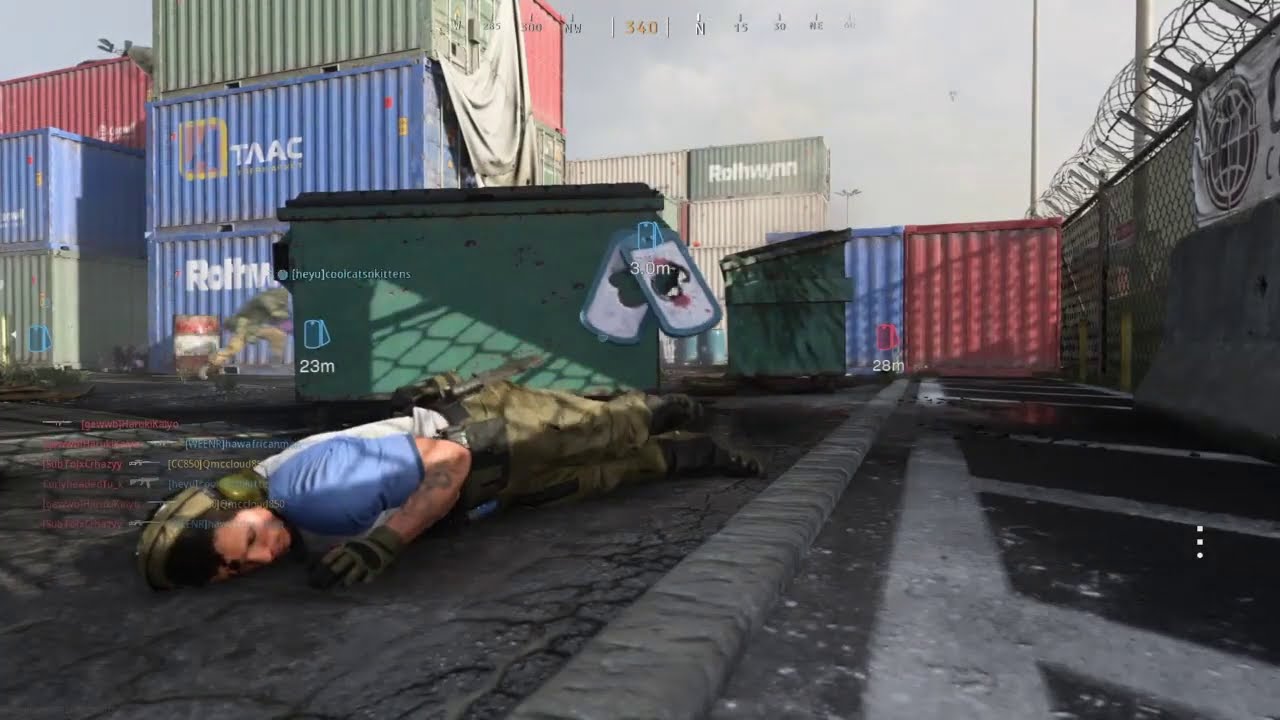The screenshot from a first-person shooter video game, likely Call of Duty, depicts an outdoor industrial area with multiple stacked shipping containers in blue, green, and red. On the asphalt ground lies a male character, possibly dead, wearing a blue t-shirt, green cargo pants, military boots, gray gloves, a black belt with a knife, and ear protection headphones. His eyes are closed and he is lying on his side. Behind him, there's a large green dumpster next to a red and blue wall. To the right, a chain-link fence topped with barbed wire borders the area. The scene is slightly overcast, with clouds visible in the background.